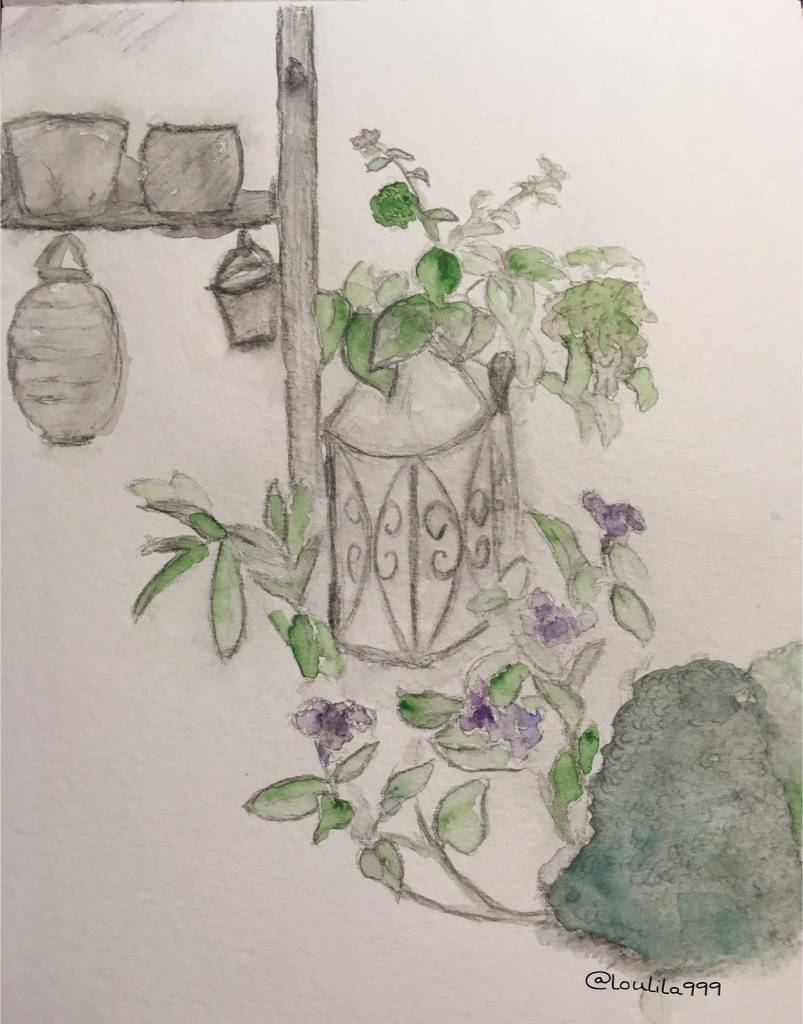This colored pencil drawing portrays a carefully crafted scene of a shelf adorned with various objects. Positioned in the upper right corner are two cups elegantly placed on the shelf. Hanging from the same shelf are two urns, each bearing intricate details. Descending from the shelf, the drawing showcases the wall, over which sits a roundish item featuring latticework along its sides and a domed top. Emerging from this ornate container is a lush branch adorned with vibrant green leaves. Below this display, to the left, rests a grayish-green rock. This rock too is sprouting greenery, but with the added charm of four branches, each boasting a delicate purple flower. The branches are accented with spade-shaped green leaves. The artwork is rendered in colored pencil, giving it a unique texture and a somewhat faded, ethereal quality.